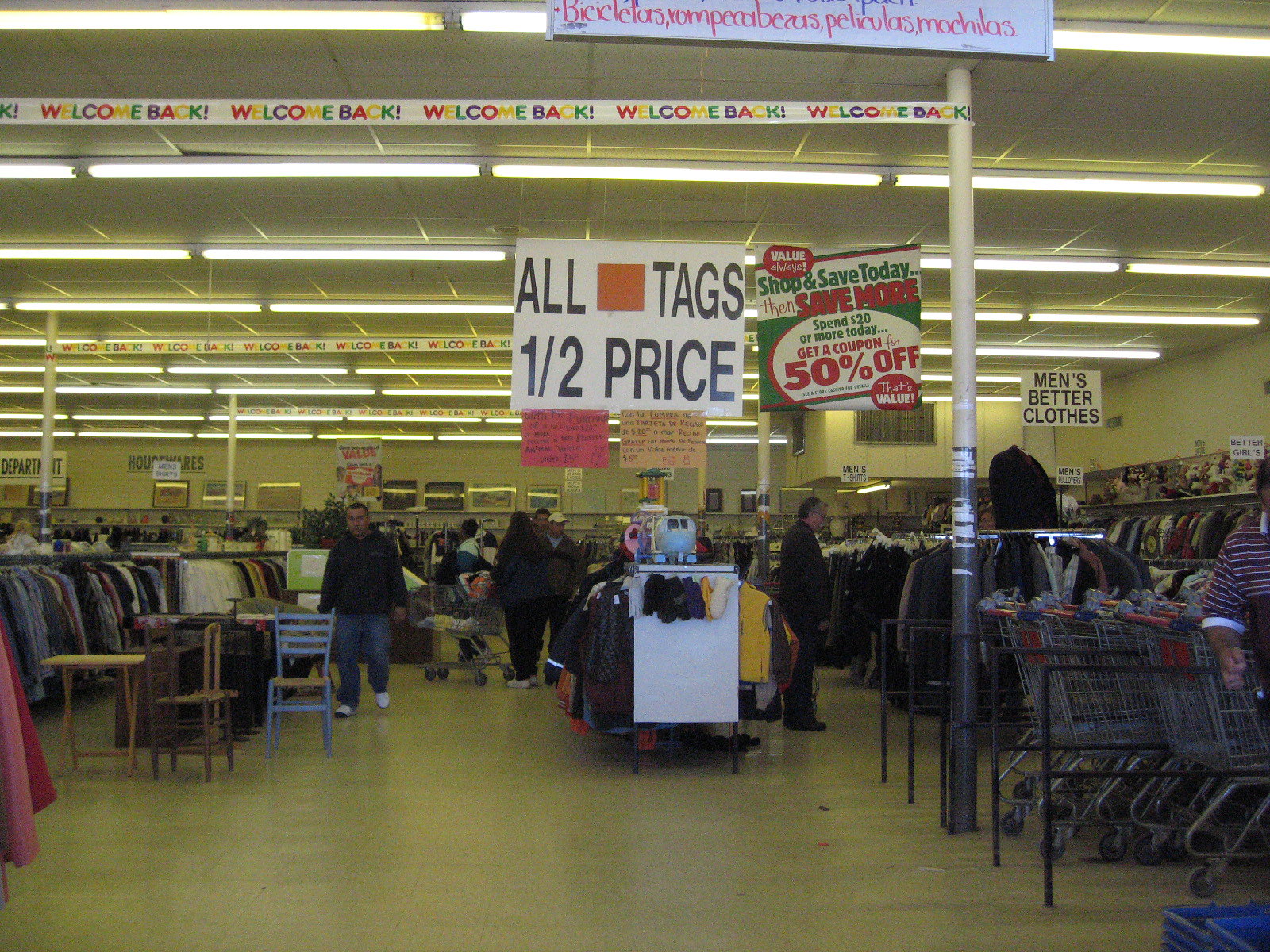The image captures the bustling interior of a discount store illuminated by rows of overhead fluorescent lights stretching across the ceiling. At the top center, a prominent white sign with vibrant pink text lists categories such as “Bicicletas,” “Rompecabezas,” “Peliculas,” and “Mochilas.” A nearby pole supports a welcoming banner with the phrase "Welcome Back" displayed in rainbow-colored letters.

Shoppers are seen perusing the various displays, with diverse clothing items—including colorful shirts and coats—hanging from long metal bars and circular racks. To the right, a line of shopping carts with distinctive red handles is neatly stacked. 

In the back right corner, the store features an area presumably filled with stuffed animals or other gifts. Various signs are scattered throughout the space, including one that reads “Men’s Better Clothes,” flanked by two small posters, one pink and the other white. Additionally, a large prominent poster announces a significant sale with the text “All Tags, One Half Price,” amidst other discount signage.